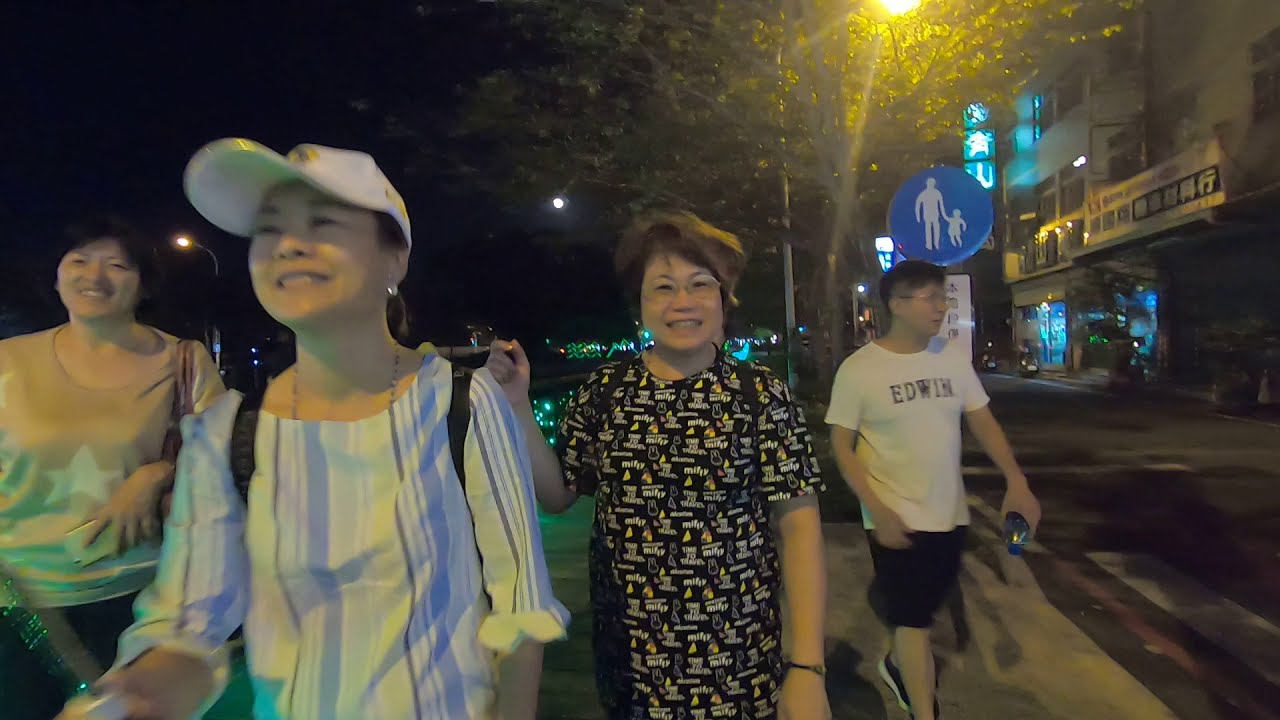This is a nighttime outdoor photograph in a city setting, featuring four individuals of Asian descent walking towards the camera on a sidewalk. The scene is illuminated by a streetlight, highlighting the group against a backdrop of dark sky and lit-up shops with foreign language signage on the right-hand side of the image.

Starting from the left, the first person is a woman with short black hair, wearing a colorful t-shirt with a prominent white star in the center. She's smiling directly at the camera and holding her phone. Next to her is a woman, possibly older, sporting a white ball cap and a long-sleeved vertical striped shirt in white, blue, and purple hues. She has a backpack on her shoulders and is facing slightly to the left, smiling up towards the corner of the frame.

In the center of the image is a middle-aged woman with short brown hair and glasses, dressed in a black dress adorned with white and yellow designs. Her right arm is raised, and she is smiling at the camera. To the far right, slightly behind the group, is a young man in a white t-shirt with the name "Edwin" printed on it, paired with black shorts and Nike shoes. He is looking off to the right, away from the group.

The brightly lit shops with Asian banners, a street sign symbolizing an adult holding a child’s hand, and a nearby tree add to the vibrant street scene captured in this photo.